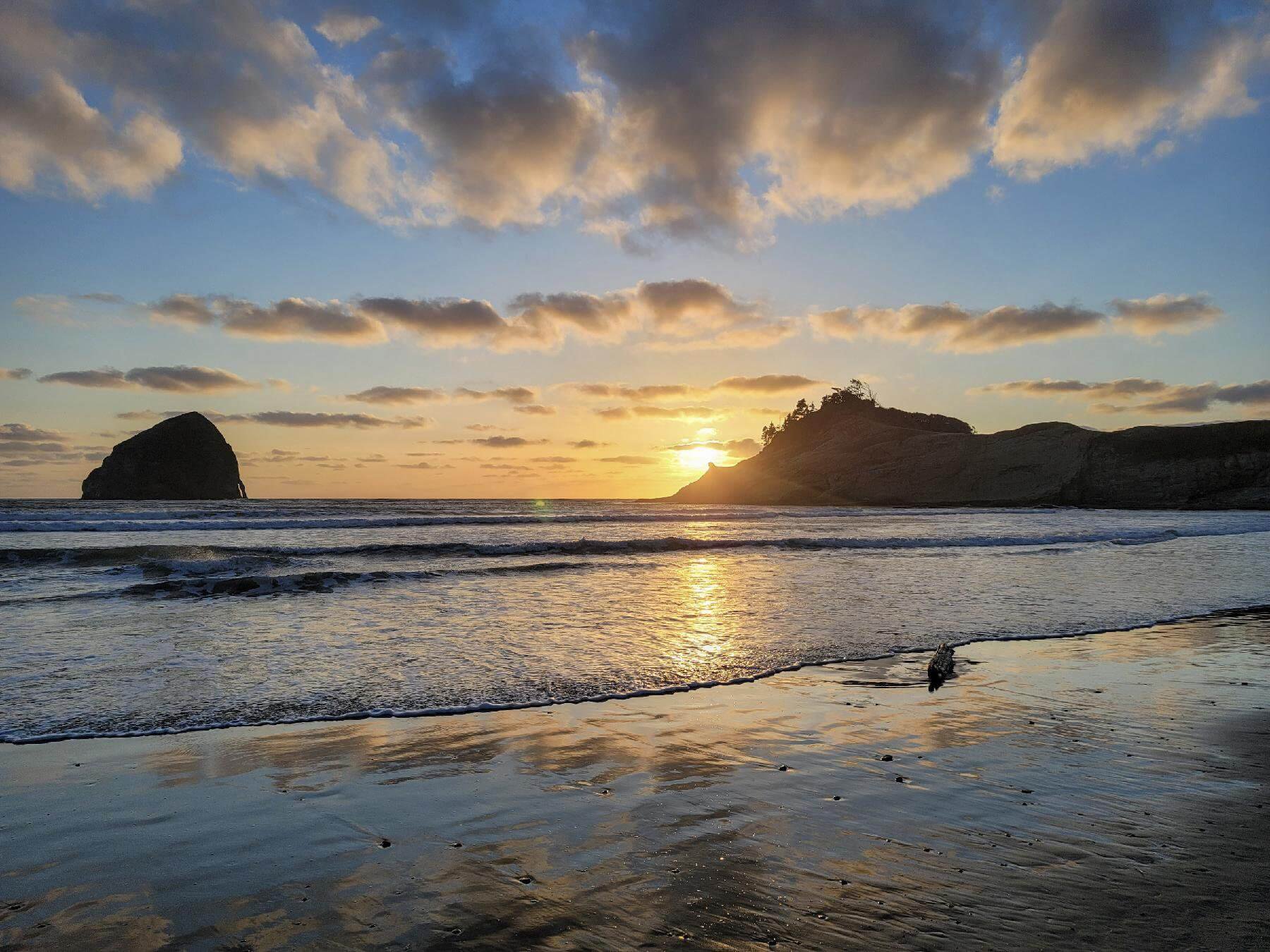This mesmerizing photograph captures the serene beauty of the Pacific Ocean at sunset, taken at the shore in Pacific City, Oregon. The image, slightly wider than it is tall, looks west over the tranquil waters as the golden sun dips below the horizon, just behind a striking land outcropping on the right. The scene is adorned with cumulus clouds streaking across a dark blue sky that lightens to a warm gradient of yellow and orange near the horizon. The glowing sun reflects off the wet sands of the beach and the calm incoming waves, which rhythmically lap at the shore. In the ocean, a prominent rock formation stands tall, adding a touch of ruggedness to the serene setting. The beach itself is hard-packed, with small pebbles scattered along its length and a piece of driftwood embedded in the sand, quietly testifying to the ocean’s timeless ebb and flow.